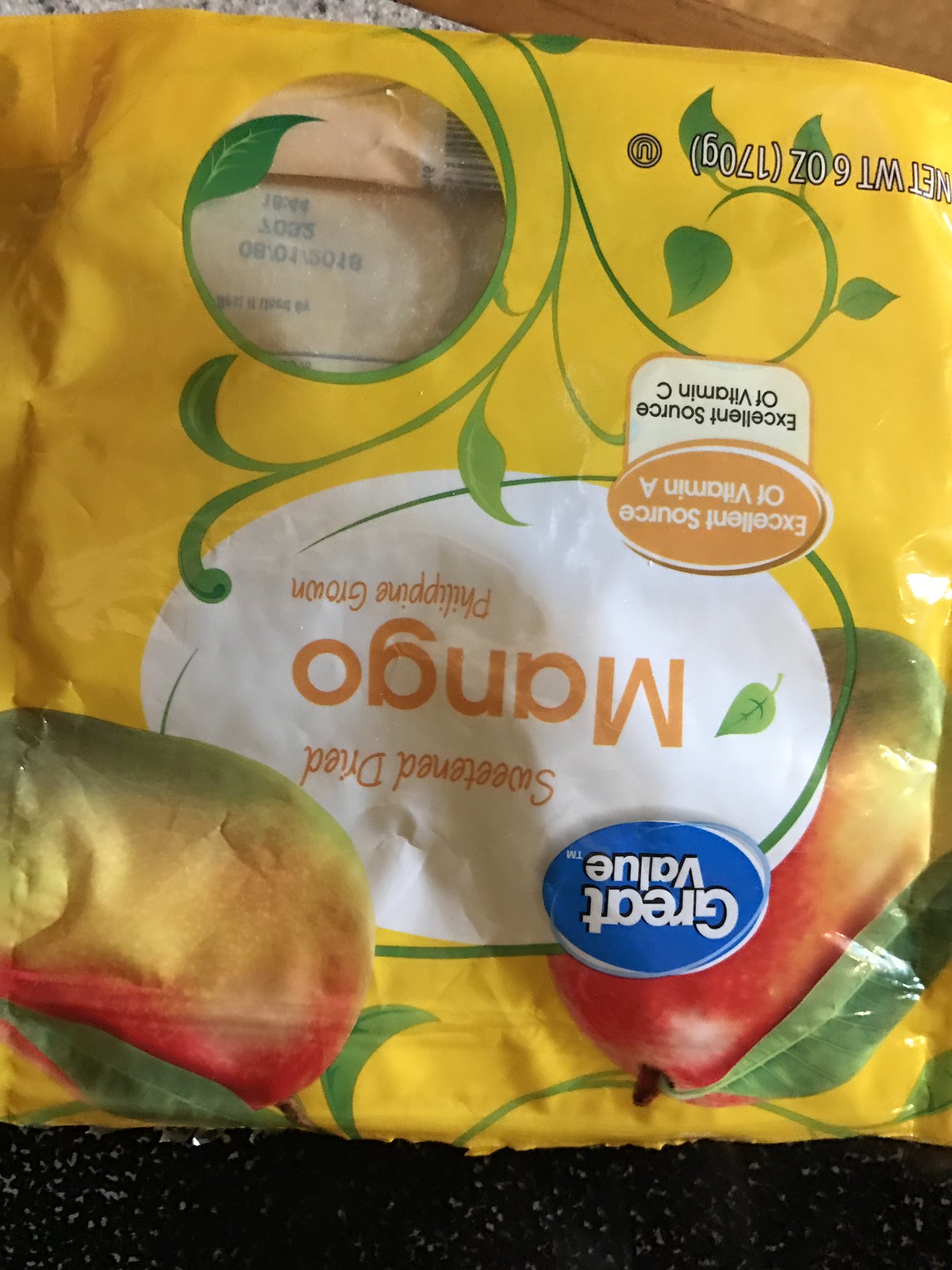The image appears to be an upside-down photograph of a bag of fruit from Walmart. The bag prominently features the "Great Value" brand logo in white text inside a blue circle. The packaging is yellow plastic and displays images of a couple of ripe mangoes. The product is labeled as "Mango, Sweetened Diced," and is noted to be "Philippine grown" or "Filipino grown." Another label on the bag highlights its nutritional benefits, indicating that it is an "Excellent source of Vitamin A" and an "Excellent source of Vitamin C." The net weight of the bag is specified as 6 ounces (170 grams).

The bag appears to have been opened, evident from its zip seal and a ragged or torn edge. The bag is resting on a dark-colored, almost black, countertop. Towards the top of the photo, part of a marble edge and a section of a wooden floor are visible.